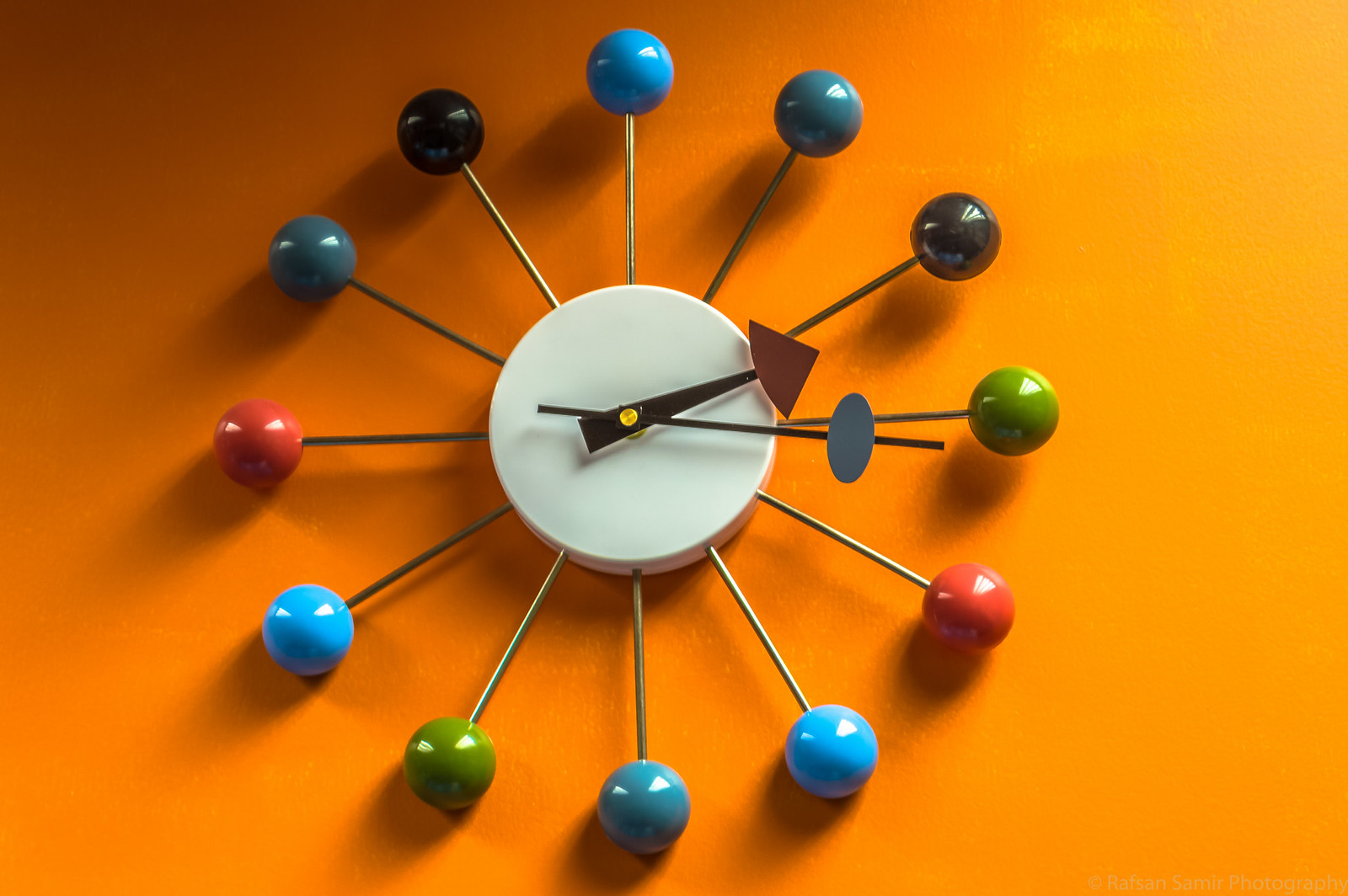This photograph features an artistic clock set against a vibrant orange background. The clock stands out with its unique face, where instead of traditional numbers, variously colored round balls mark the hours. These balls transition through a spectrum of colors, ranging from light blue to dark blue, black, green, and red. Each ball is connected to a central white hub by sleek metal rods, creating a visually striking and modern design. The clock hands add to the artistry; both are black, but the hour hand is distinguished by a red pie-shaped pointer, while the minute hand features a blue oval-shaped pointer. This blend of bold colors and inventive design makes the clock a captivating focal point in the image.